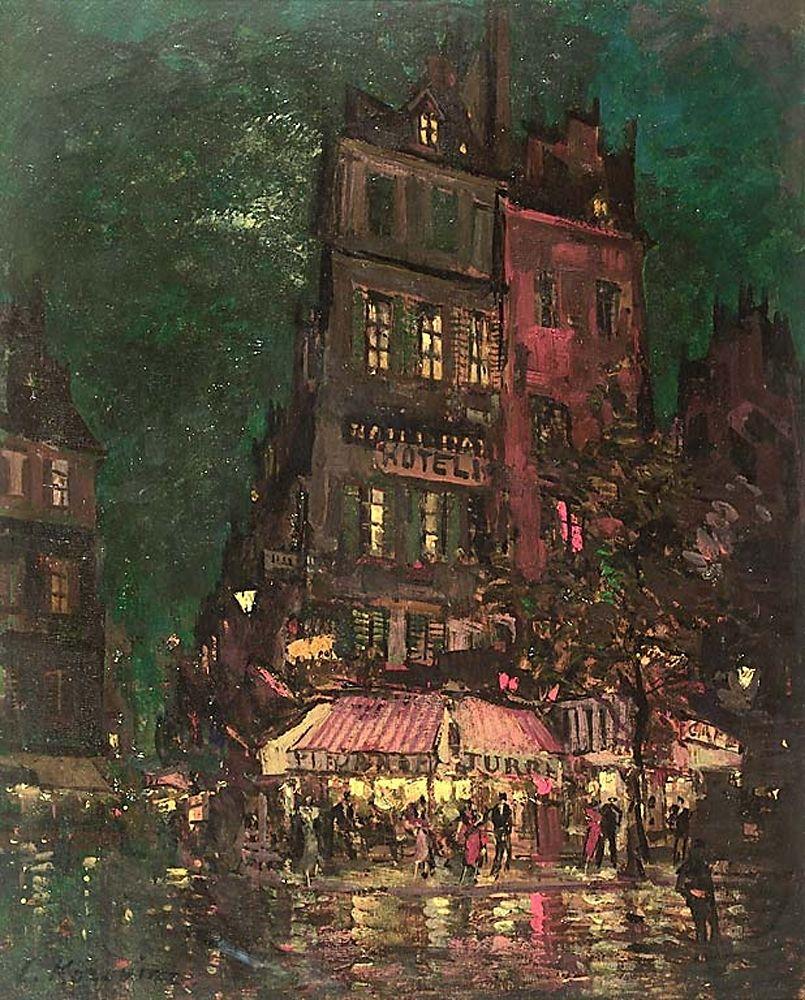This impressionist painting, likely inspired by turn-of-the-century Paris, features a bustling night scene in portrait orientation, with an aura of elegance and style. The central focus is a grand hotel complex comprising two closely adjoined buildings, each standing approximately five to six stories tall. The building on the left is a dark brown structure with arched rooftops, adorned with a sign that reads "PORTAL," and illuminated windows casting a yellow glow. The adjacent building to the right is slightly shorter and painted in a reddish hue, contributing to the vivid contrast.

Both buildings have warmly lit awnings on the ground floor, underneath which several elegantly dressed individuals—some in dresses, others in tuxes or top coats—are seen mingling and shopping. The wet pavement below captures the reflections from the awnings and windows, enhancing the scene's shimmering effect. The dark green sky overhead completes the nocturnal ambiance, further accentuated by the slanted rooftops and dormer windows evocative of the French left bank style.

This detailed scene is signed by the painter in the bottom left corner, adding a personal touch to this evocative and stylish representation of a formal, lively night in an urban street.